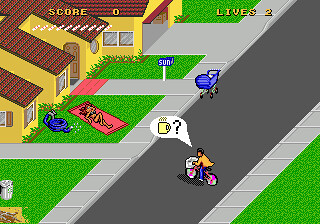The image depicts a screenshot from a colorful computer game. At the top of the screen, there's a score display in bold yellow text, showing "SCORE" alongside a value of "0." To the right, the word "LIVES," also in yellow, indicates the player has two lives remaining.

The scene in the game features a suburban neighborhood with lush green grass yards. A gray road cuts diagonally through the center of the image, flanked by silver sidewalks. In the middle of the road, a character on a bicycle is facing one of the houses. The houses are painted yellow with red shutters and topped with red roofs.

In the foreground, a woman is sunbathing on a red towel on her lawn. Nearby, a blue garden hose is coiled on the grass. A blue baby carriage stands by the side of the street. Above the bicyclist's head, a text box with a question mark hovers, suggesting an element of inquiry or interaction within the game.